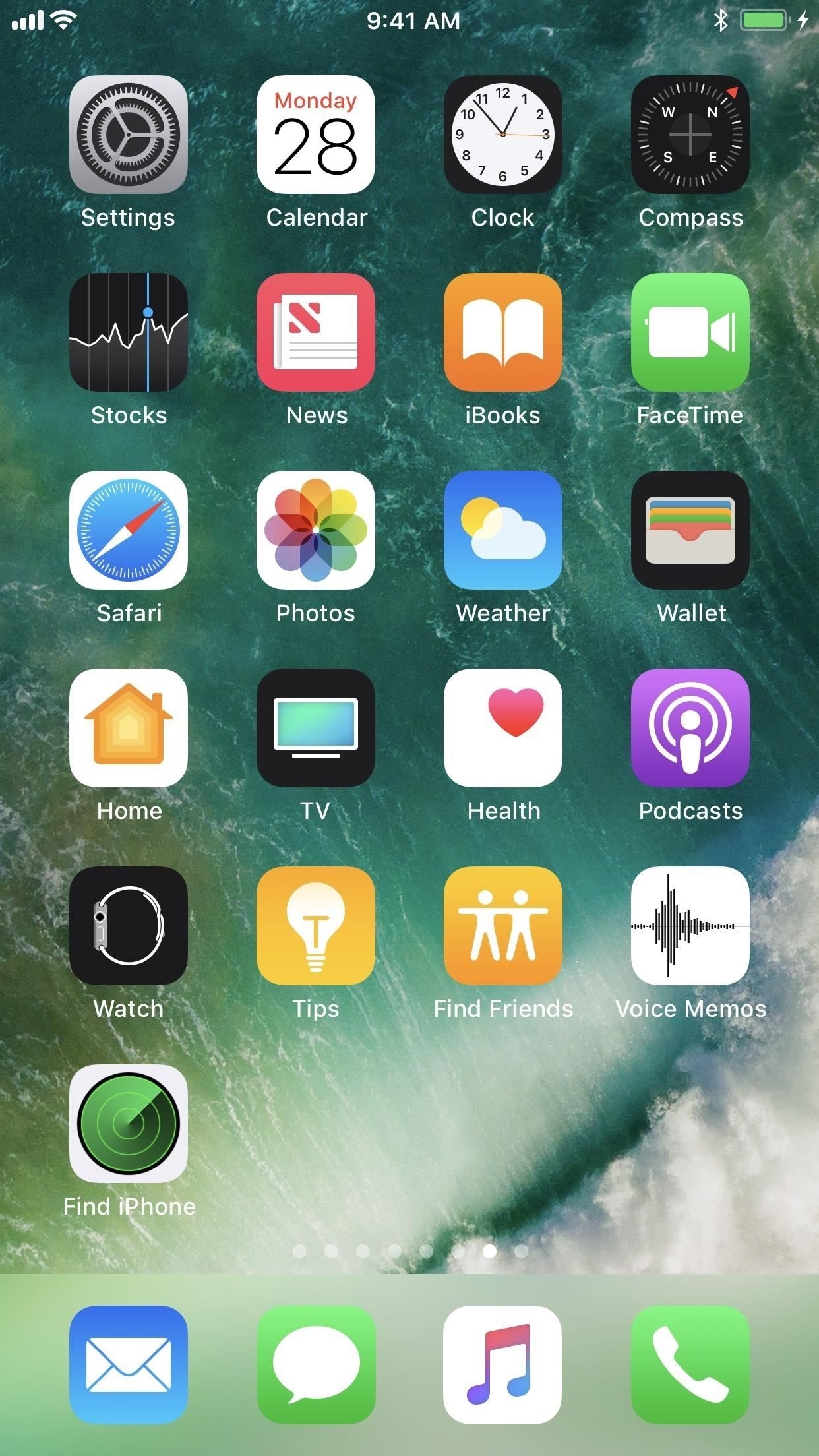The image showcases a smartphone screen with a backdrop of serene bluish water. At the top of the screen, there are various status indicators including Wi-Fi signal strength, battery percentage, and Bluetooth connectivity.

The screen is populated with a multitude of app icons arranged in a grid format:
1. **Settings**: Represented by a grey gear icon.
2. **Calendar**: Featuring the date "Monday the 28th".
3. **Clock**: Depicted with an analog clock face showing all 12 hours.
4. **Compass**: Displaying the cardinal directions (N, S, E, W) on a dark background.
5. **Stocks**: Indicative of a financial app.
6. **News**: Illustrated with a newspaper icon.
7. **iBooks**: Represented by a book icon.
8. **FaceTime**: Shown with a green and white camera icon.
9. **Safari**: Featuring a circular compass-like icon.
10. **Photos**: Likely to be shown with an image-related icon.
11. **Weather**: Depicted with a cloud and sun.
12. **Wallet**: Indicative of a financial management app.
13. **Home**: Referring to a home automation setup.
14. **TV**: Symbolic of a media streaming app.
15. **Health**: Represented by a white and pink heart icon.
16. **Podcasts**: Highlighted with a purple background and icon.
17. **Watch**: For managing smartwatch settings.
18. **Tips**: Likely shown with a light bulb icon.
19. **Find Friends**: Suggesting a location-sharing app.
20. **Voice Memos**: Depicted by a waveform or microphone.
21. **Find iPhone**: Represented by a green radar icon.
22. **Mail**: Illustrated with a white envelope on a blue background.
23. **Messages**: Typical speech bubble icon.
24. **Music**: Shown with a musical note icon.
25. **Phone**: Displayed with a white phone icon on a green background.

The wallpaper sets a tranquil tone with its watery, bluish hues. This organized arrangement of icons on the smartphone screen provides a comprehensive overview of its apps and functionalities.